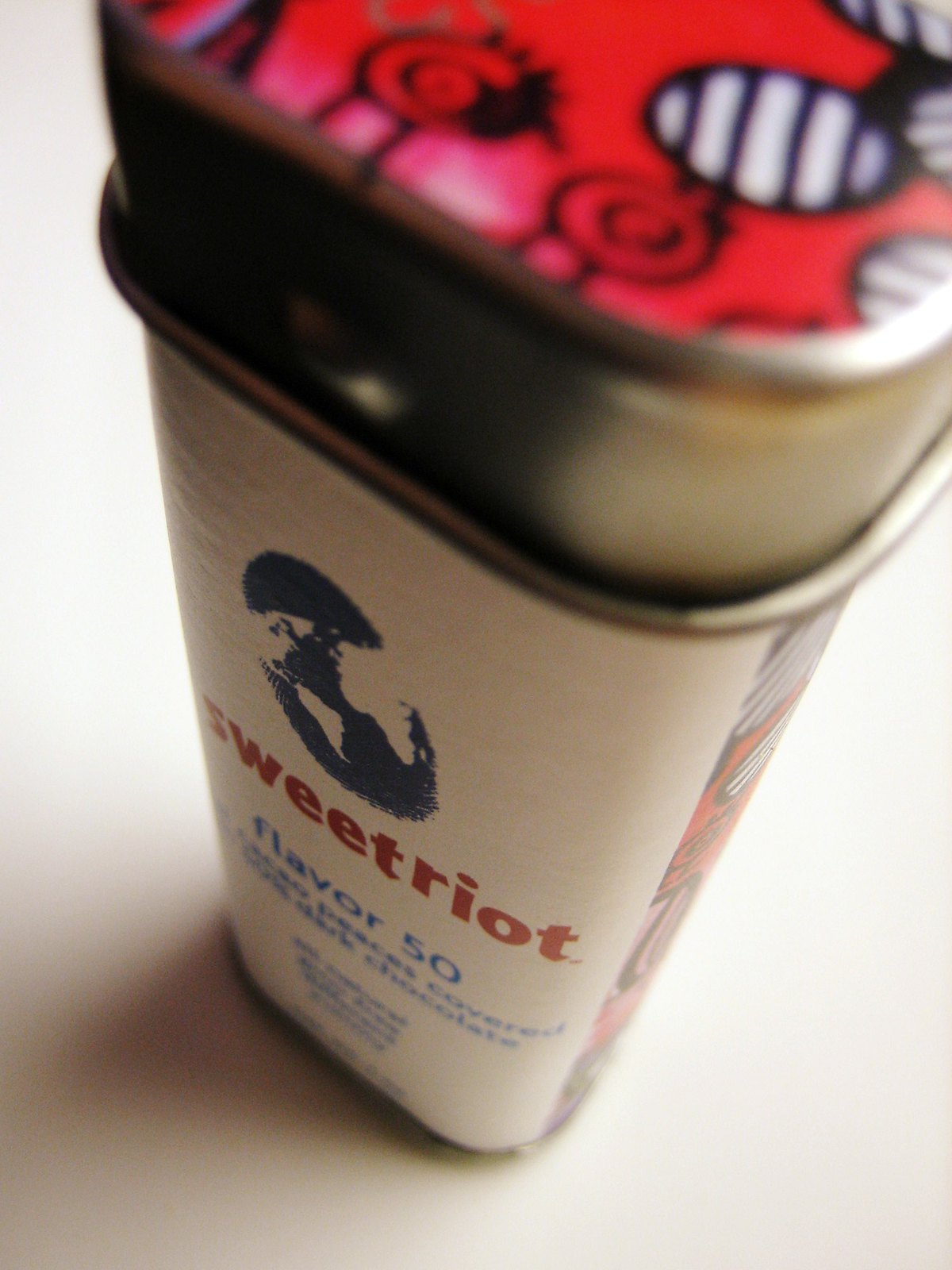The photograph is an indoor, close-up image taken from a high vantage point, looking down at the top of a vertically-oriented, rectangular, metal tin container with a square base. The container features a silver cap adorned with a red circular pattern that extends slightly around its top edge. The tin sits on a white surface, casting a soft shadow to the left due to lighting from the upper right.

The tin's front bears a white label featuring a blue globe logo, which combines a world map with a fingerprint design. The landmasses depicted include the Americas, Europe, and Africa. Below the globe, in lowercase red letters, is the brand name "Sweet Riot." Further below, in smaller blue letters, it reads "Flavor 50." There are additional lines of text beneath this, but they are not legible in the image. Aside from the label’s text, there are no other discernible markings or inscriptions visible. The precise purpose of the container is not clear, though it is suggested to be some sort of flavor additive or spice.